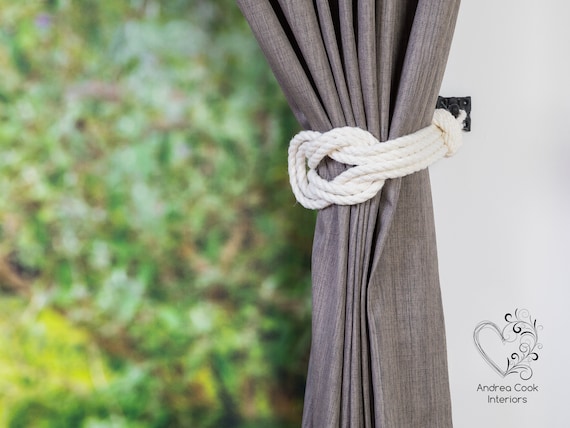This color photograph appears to be an advertisement for Andrea Cook Interiors. It features a sophisticated gray linen curtain, elegantly pleated and tied back with a decorative white rope in a nautical, figure-eight knot. The curtain is anchored to the wall with a wrought iron or rubbed bronze hook, firmly mounted on the white wall to the right. Beneath this hook, in the bottom right corner, lies a black and white logo—a heart with curling vines on the right side and the text "Andrea Cook Interiors" beneath it. The left side of the image depicts an out-of-focus window view, revealing a palette of green, brown, and yellow hues, suggesting an external garden scene but lacking any clear detail. This composition showcases both the refined interior curtain design and hints at a tranquil outdoor environment, creating a balanced and inviting promotional image.